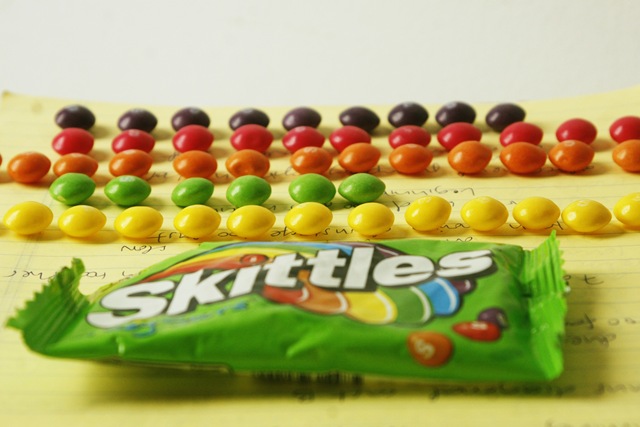The image captures a meticulously arranged display of Skittles candy on a yellow piece of loose-leaf paper with pen writing, though the text is unreadable. The background is a grayish, off-white color occupying the top 20-25% of the photo, while the yellow paper takes up the remaining bottom section. The Skittles are organized in five horizontal rows by color: the top row features dark purple or brown Skittles, followed by red, then orange, and next a shorter row of green Skittles that only spans half the width of the others. The bottom row consists of yellow Skittles. Beneath these rows is a ripped-open green plastic Skittles wrapper, prominently displaying white lettering and colorful Skittles graphics, with a rainbow extending from the word "Skittles." The image is likely set on a desk inside someone's house.